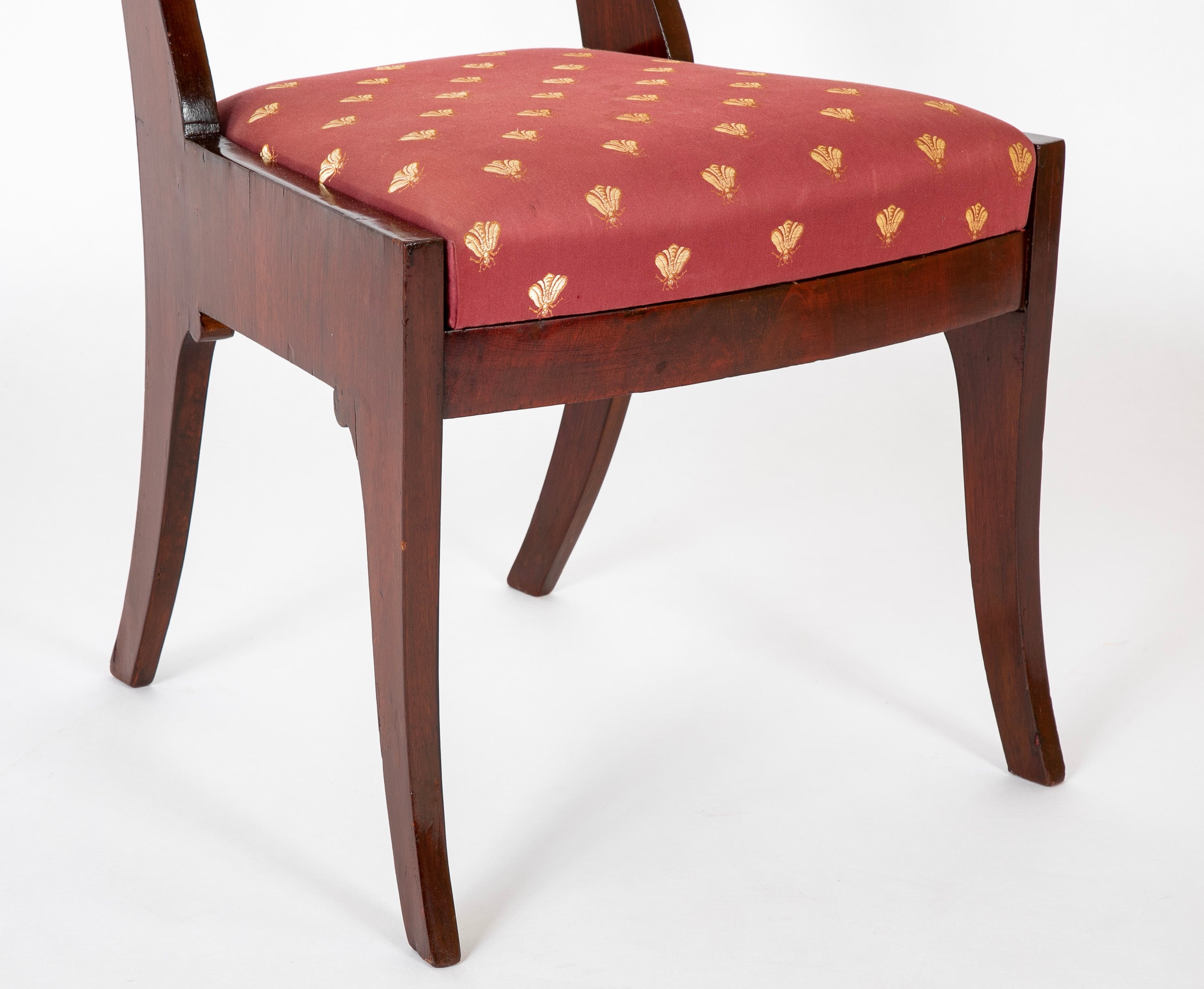The image depicts the lower half of a traditional, elegant dining room chair made of mahogany-colored wood, set against an all-white background, giving it the illusion of floating in space. The chair features a detailed upright wood structure and outspread, sturdy legs. Its seat cushion, in a vibrant orangey-red or tangerine hue, is adorned with intricate leaf and wheat motifs in a gold or yellow color pattern, which repeat about an inch apart across the cushion. The chair has an old-fashioned aesthetic, reminiscent of something that might be found in a museum. While the high back of the chair is not visible in the photograph, the craftsmanship and rich design elements suggest it is both a functional and a visually appealing piece of furniture.